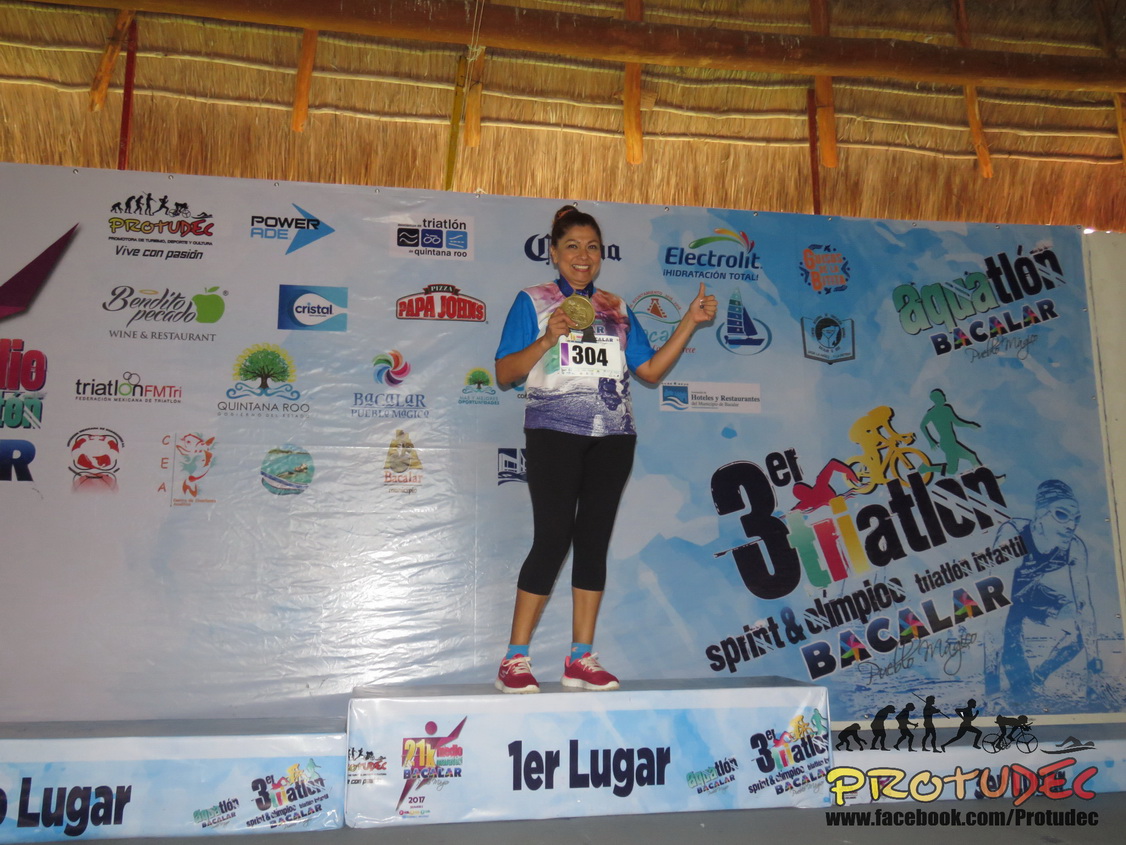The image depicts a triumphant woman who has just won a triathlon, standing on the first-place podium marked "1er Lugar." She is indoors within a straw hut, set against a large white backdrop adorned with numerous sponsor logos such as Papa John's, Corona, Electrolit, Powerade, Crystal, and Quintana Roo. The backdrop prominently features the event title "3er Triathlon," illustrated with colorful icons representing swimming, bicycling, and running, and includes mentions of "sprint" and "Dimpio triathlon."

Clad in a jersey with blue sleeves and green-and-red design, black capri pants, red sneakers, and light blue socks, the woman bears a chest tag denoting her race number as 304. Her dark hair frames a smiling face, and she holds a large gold medal in her right hand while giving a thumbs-up with her left. The podium she stands on is the tallest of three, with no one occupying the lower second and third place podiums. The scene is filled with an array of sponsor logos like "Rendito Picado Wine and Restaurant," "Protodeck," and more, with detailed illustrations such as a green apple and tree, contributing to the celebratory atmosphere of her victory.